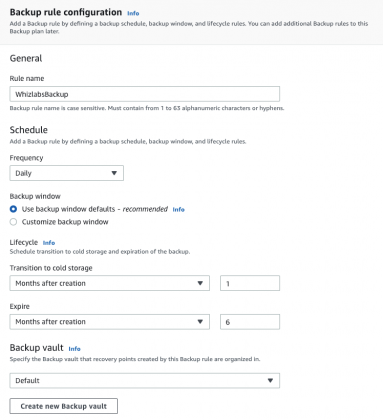The image depicts a user interface on a white background, designed for setting up a backup rule. At the top, there's a gray banner featuring the text "Backup Rule Configuration" in black print. Adjacent to it, in blue font, is the word "Info," which appears to be a clickable hyperlink for additional information.

Below the banner, a gray text block reads: "Add a backup rule by defining a backup schedule, backup window, and lifecycle rules. You can add additional backup rules to this backup plan later."

Further down, the interface displays a section labeled "General Rule Name" with a text box containing "Wyslabs backup." Instructions indicate that the backup rule name is case-sensitive and must consist of 1 to 63 alphanumeric characters or hyphens.

The subsequent fields allow for the detailed configuration of the backup schedule:

- **Schedule**: Includes a dropdown menu with the option "Daily" selected by default. A descriptive note reads: "Add a backup rule by defining backup schedule, backup window, and lifecycle rules."
- **Backup Window**: Offers three options: "Use backup window's default," "Recommended," and "Custom backup window," with the default option being selected.
- **Lifecycle**: Specifies settings for the transition to cold storage and expiration of the backup. The transitions are set to move to cold storage one month after creation and to expire six months after creation.
- **Backup Vault**: The default backup vault is selected, with the option to create a new backup vault if desired.

This detailed configuration panel allows users to meticulously organize and manage their backup rules and lifecycle policies.